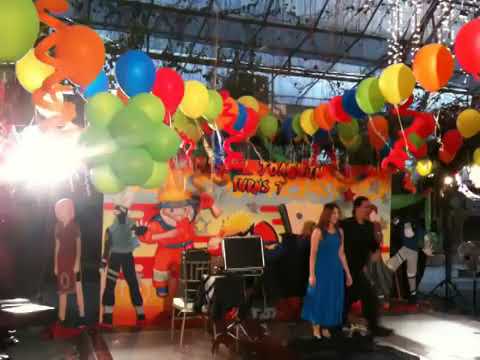In this vibrant image, a lively celebration, likely a birthday party, is captured on a plain stage adorned with colorful decorations. Dominating the scene are numerous bright balloons in shades of orange, green, yellow, blue, and red, creating a festive canopy above. Across the top, there are streamers interwoven with rainbow-colored balloons, enhancing the cheerful atmosphere. At the center of the stage, a woman in a long blue dress with dark brown hair stands beside a man dressed entirely in black, from his shirt to his shoes, with matching black hair. Together, they appear to be the focus of the event, possibly performing. Behind them, a vivid backdrop features spray-painted cartoon characters, including the recognizable Naruto, and it seems to announce someone turning seven. Additionally, a table with a black briefcase with a metal trim is placed behind them, adding to the scene's setup. The joyous environment suggests a celebration filled with laughter and color.